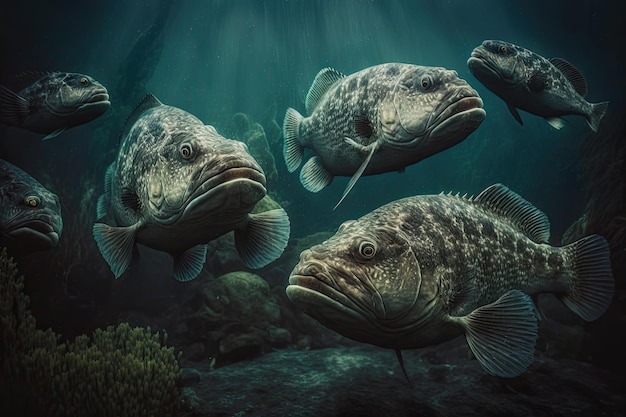This underwater scene showcases a group of grouper-like fish, likely captured in a photograph or a meticulously designed computer image. All the fish feature similar characteristics: frowning, lip-like mouths, large knotted heads, and a mottled gray color with a bluish tint. Their bodies are stocky with small fan-like fins and tails. The fish are of various sizes, with smaller ones appearing further away due to perspective. The dark, murky underwater setting is illuminated lightly from above, transitioning to deeper greens and teals in the background. The scene includes some aquatic elements like kelp and rocks on the ocean floor, enhancing the naturalistic feel. The grouper-like fish exhibit slight color variations with subtle white speckles across their uneven skin, giving them a chameleon-like adaptability to blend with their environment.